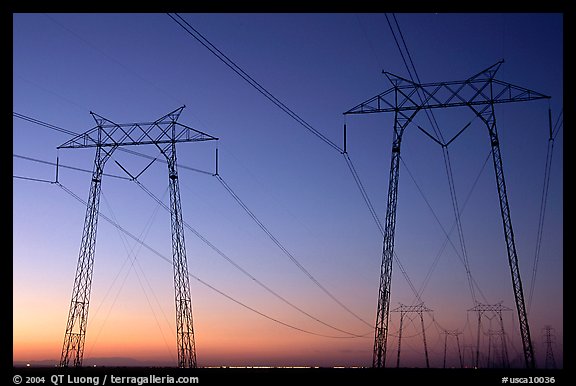The photograph showcases a vast expanse of power lines and electrical towers captured during dusk. Prominently in the foreground, two metal towers rise approximately 150 feet, one positioned to the left and the other to the right. Each tower features three extended power lines, running horizontally, connected to similarly robust towers that recede into the background, demonstrating the extensive reach of the power grid. The towers are designed with unique structures at the top to bear the weight and dynamic tension of the wires.

The sky transitions from a deep evening blue at the top to a lighter blue towards the horizon, with the setting sun casting a pale yellow, pale orange, and red-orange glow, creating a striking contrast against the silhouetted towers and wires. The photograph exudes a serene, end-of-day atmosphere with the sun descending slowly, illuminating the scene with warm hues.

At the bottom of the image, a black border frames the photograph. The left side of the border bears the text, "Copyright 2004, QT Luong, TerraGalleria.com," while the bottom right corner displays "#USCA10036" in small white font.

This detailed, beautifully composed image not only captures the intricate infrastructure of the power system but also melds it seamlessly with the natural beauty of a sunset sky.